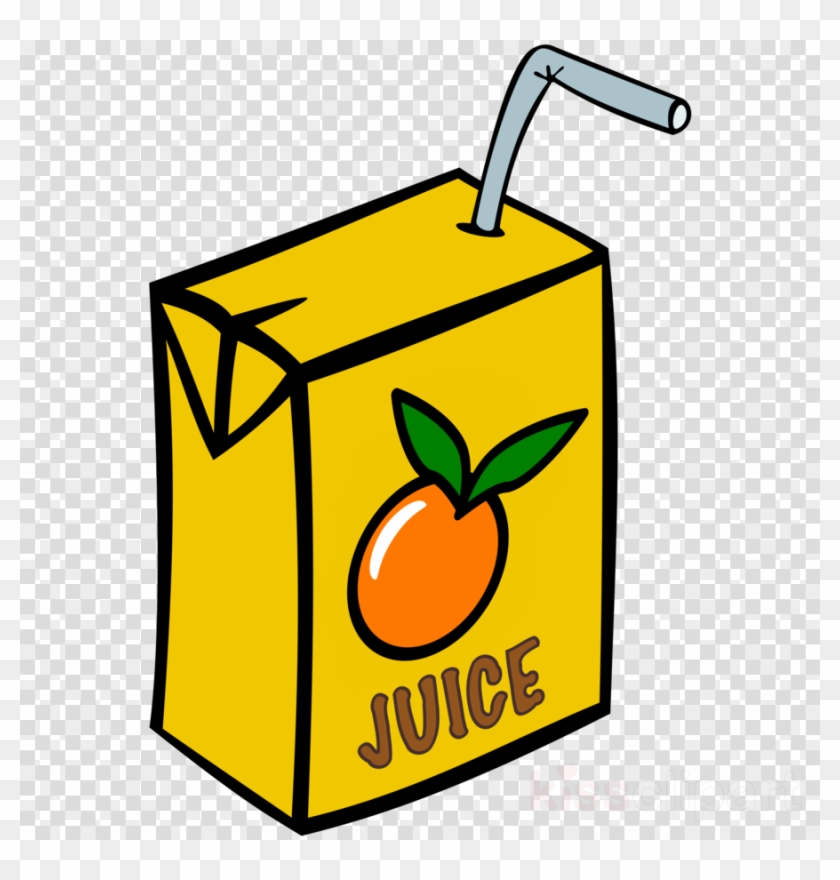This is an intricate 3D cartoon illustration of a yellow-orange juice box, set against a detailed background of interconnected purple and white checkerboard squares. The checkered pattern consists of smaller squares forming a woven texture, with a double-lined border of lighter purple and white squares along the top, bottom, left, and right edges. The juice box is depicted facing forward and slightly to the right, highlighted by a thick black outline. On the front of the box, there's a round orange graphic with two green leaves and a white streak suggesting sunlight. Below the orange, the word “JUICE” is prominently displayed in large brown capital letters. The juice box also features a small hole in the top right corner, with a gray or light blue straw bent at a 90-degree angle, extending outward and slightly to the right.